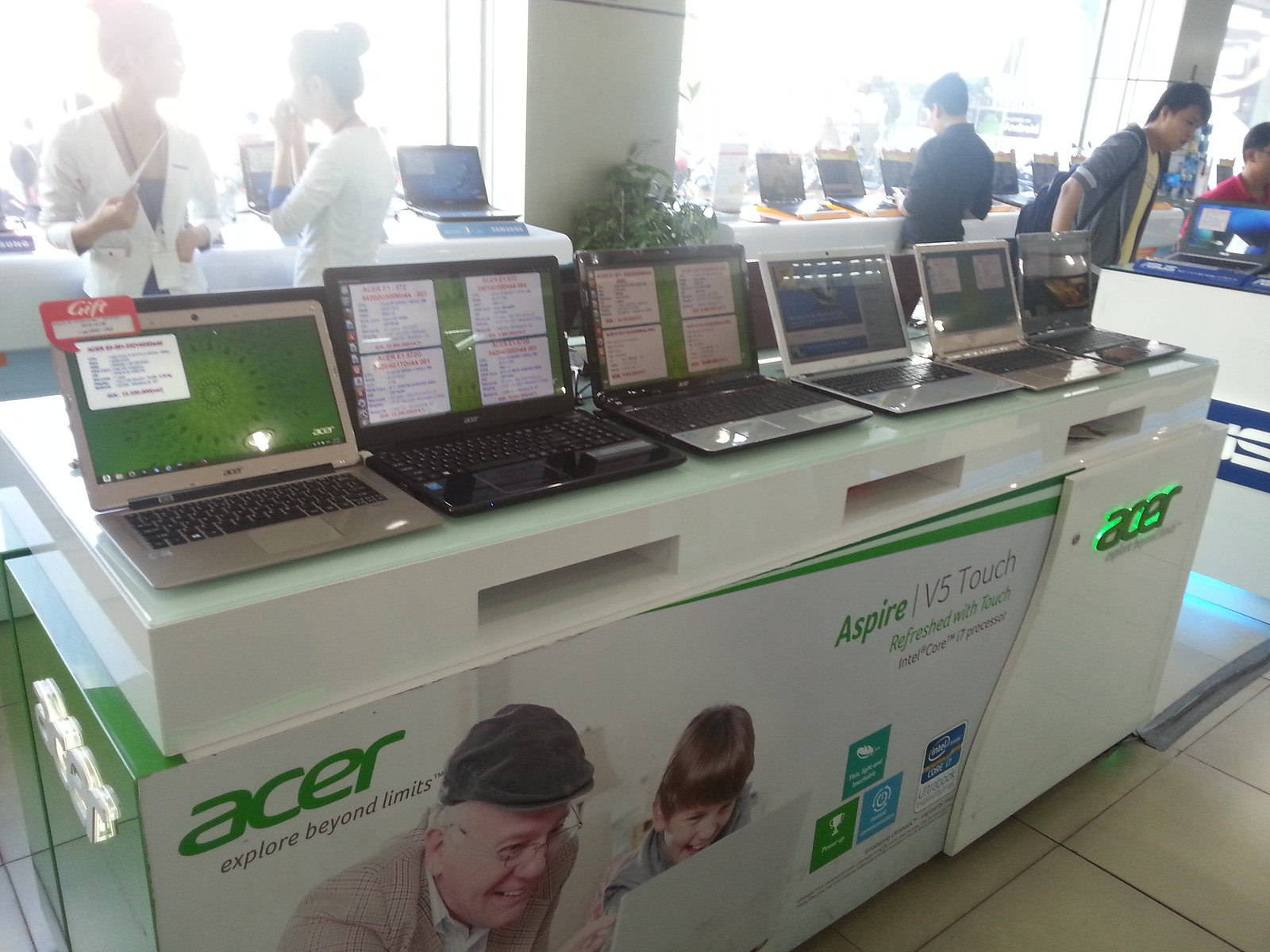This detailed photograph showcases a vibrant Acer product display within a retail store or a product expo. Central to the scene is a tall, rectangular white platform adorned with six laptops of varying colors, including gray, black, and silver. Four of the six laptops have green screens, resembling the green shade of the prominently featured ACER logo, while one laptop seems to be turned off and another displays different content. A notable laptop on the far left corner is marked with a red "GIFT" tag.

Below the laptops, attached to the side of the platform, is a large sign with the ACER logo, the slogan "Explore Beyond Limits," and an image of two smiling individuals using a laptop, specifically highlighting the Aspire V5 Touch model. Next to this sign on the right edge of the platform, a lit green ACER logo adds a vibrant touch.

The surrounding floor is covered in white square tile-style flooring, and in the distance, the store's bright white windows illuminate the space. Two women, possibly staff or sales assistants, are seen behind the display, dressed in white suit coats or cardigans with blue undershirts and black lanyards, one holding a document and the other with her hands near her face. Additional rows of laptops from various vendors are visible in the background, adding depth to the busy retail atmosphere. A house plant in the center of the image provides a touch of greenery, and the faint, partially visible blue Asus logo marks the far right edge of the frame.